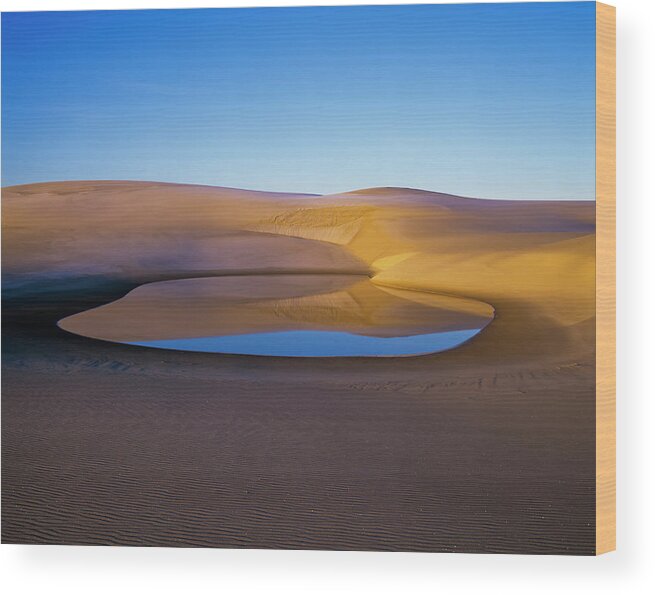In a beautifully detailed desert landscape, this piece—either a painting or a photograph on wood—captures the mesmerizing simplicity of sand dunes beneath a crystal-clear blue sky. The horizon is divided into two distinct sections: the lower two-thirds show gently rolling, low-lying dunes, while the upper third showcases an expansive, unclouded sky that deepens in blue towards the top and lightens near the dunes. Centrally positioned is an oblong and still body of water, so reflective it's almost mirror-like, capturing the surrounding dunes and sky within its depths. This small pond enhances the interplay of colors, turning the nearby sand into a darker brown where wetness meets dryness. Detailed wind patterns trace across the sand, adding subtle texture to the landscape. Overall, the image conveys a serene and timeless desert scene, devoid of vegetation or human presence, emphasizing the natural beauty and patterns formed by the elements.